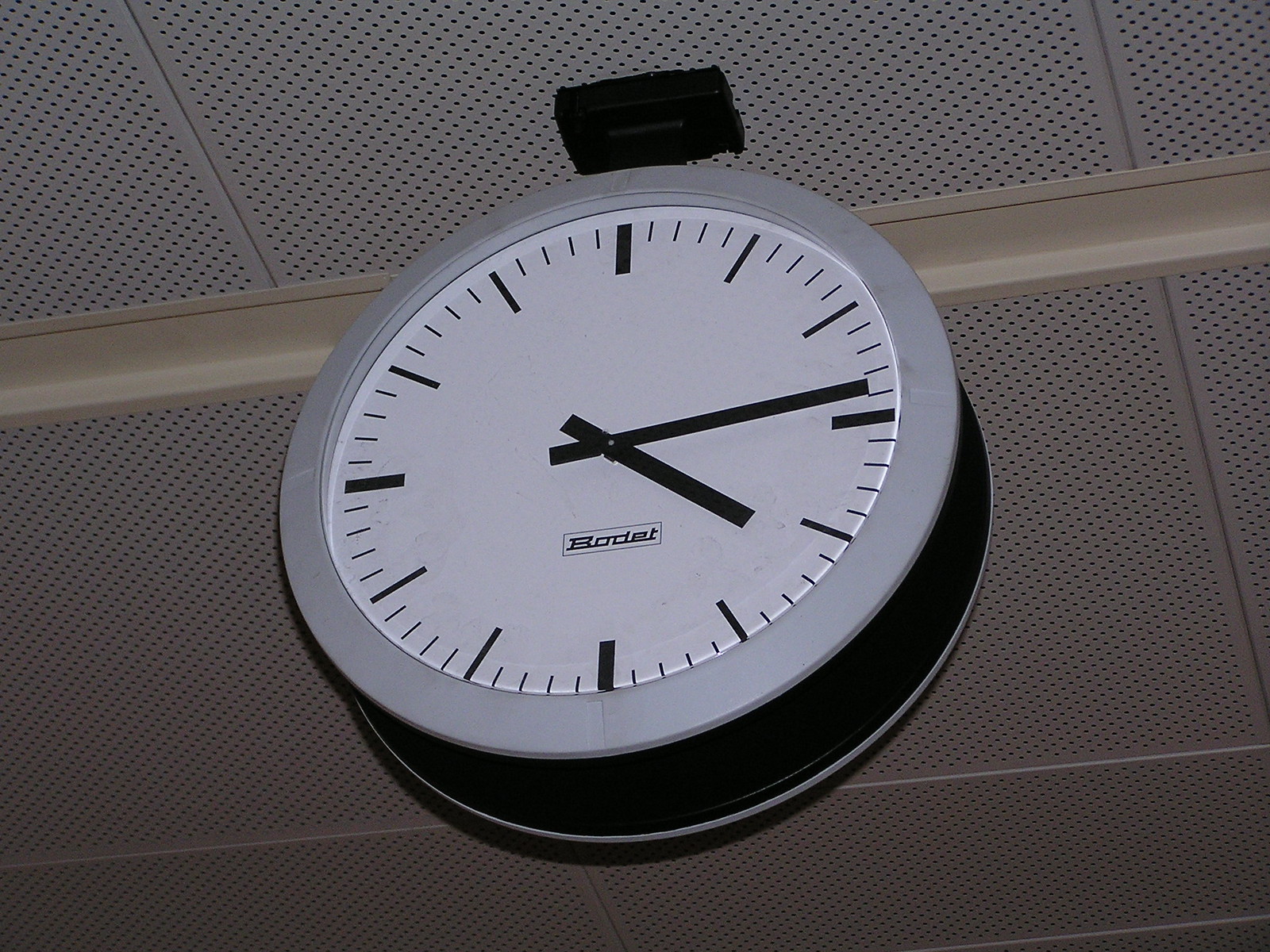The image features a clock suspended from a ceiling constructed of metal mesh. Detailed crown molding is visible at the top of the scene. The clock itself stands out with its almost surreal appearance. It has a black outer casing and a gray trim encircling its white face. Prominently displayed on the face is the brand name "BODET." The clock features black hour and minute hands but lacks a second hand. Instead of traditional numbers, the clock face is marked with simple lines, with slightly darker lines indicating the 12, 3, 6, and 9 positions, and lighter lines marking the hours in between. The clock is mounted against a wall that is not fully described but adds to the contextual ambiance of the setting.